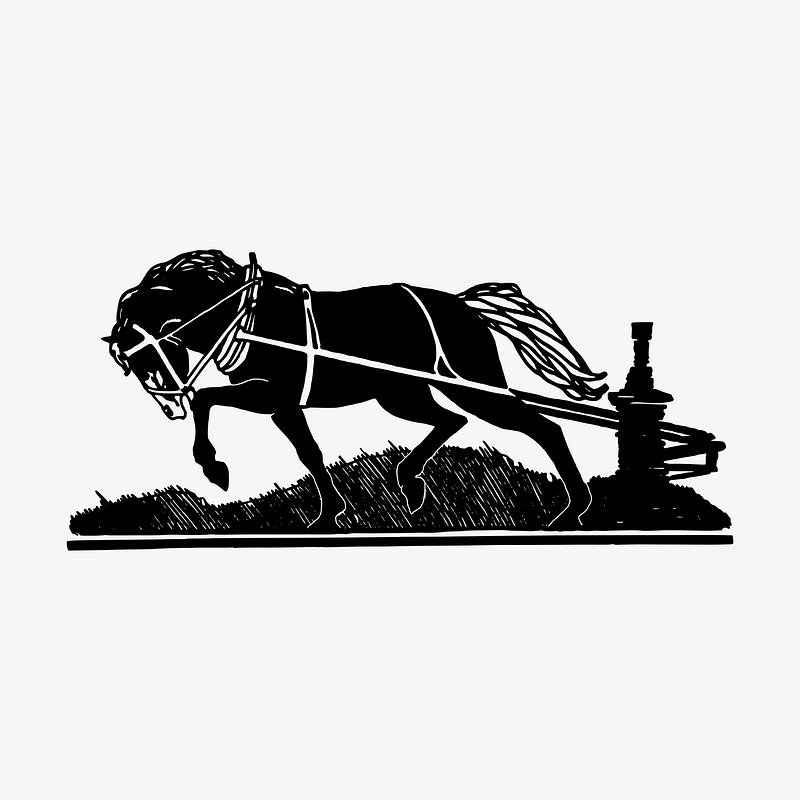In a detailed black and white silhouette artwork set against a very pale beige background, a fully harnessed black horse with a distinctive white mane and muzzle is depicted straining to pull a stone structure embedded in the ground. The horse, clearly illustrated with defined bridle and harness, appears determined yet unable to move the heavy object it is tethered to. Below the horse, delicate black strokes symbolize patches of grass, adding a touch of natural texture to the scene. The overall composition captures the intense effort of the horse, poised in mid-struggle, unable to break free from what binds it.